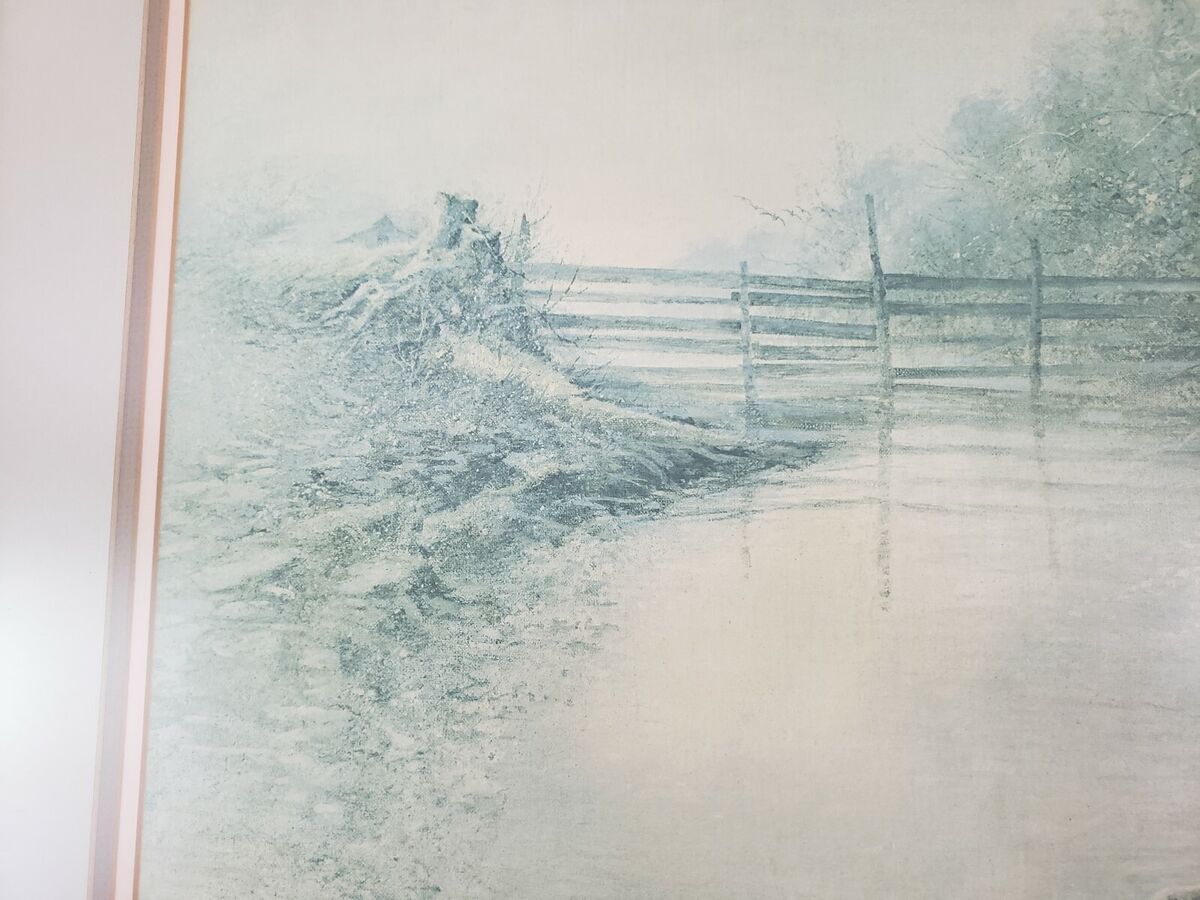The image depicts a partially faded, predominantly monochromatic painting, framed in a light brown or beige frame visible on the left side, set against a gray wall. The painting captures a serene landscape featuring a meandering creek or pond with a reflective surface, flanked by a wooden fence that runs across the water, creating a barrier. On the left side of the water, there is some land characterized by rocks, mud, or sand, while the right side reveals several trees growing beyond the fence. In the background, additional foliage, possibly including a barn, and trees add depth to the scene. The overall color palette of the painting leans towards shades of gray with hints of green, contributing to its faded, vintage quality.